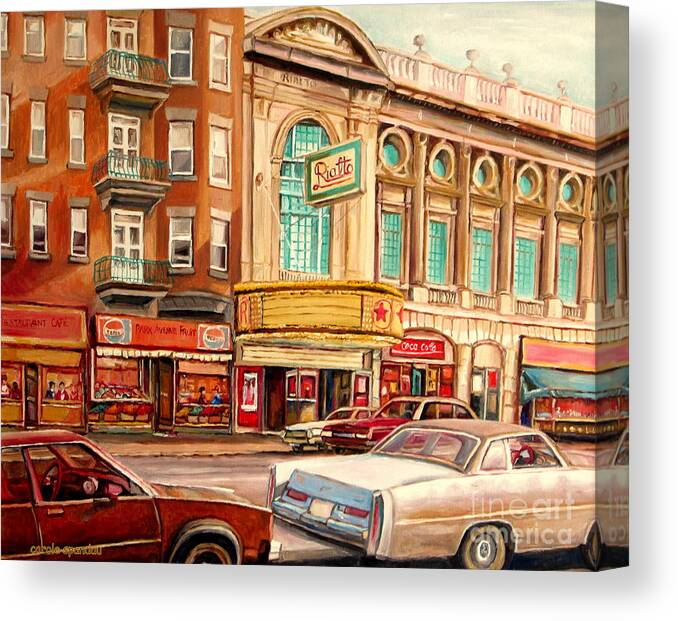**Caption:**
This detailed illustration appears to be a realistic oil painting of a vintage downtown area from the 60s or 70s. Dominating the scene is a street stretching across the bottom of the painting, with boxy, long-bodied cars typical of the era, such as Pontiacs and Buicks. Two cars—one red and one white—are parked in the foreground, while two others drive down the center of the street.

On the left side, we see a brick building with at least four stories, featuring balconies and housing shops or cafes on the first floor. Notably, there's a restaurant or cafe, and a convenience store marked with Pepsi logos. The architecture transitions to more opulent designs on the right, where the Rialto Theater stands. The theater, with its stone construction, boasts decorative elements, including a marquee and large, blue arched windows spanning two stories. This area likely features commercial spaces on the ground floor, with residential or additional commercial usage above. The entire scene exudes an old-timey, nostalgic charm, reminiscent of a bygone era.